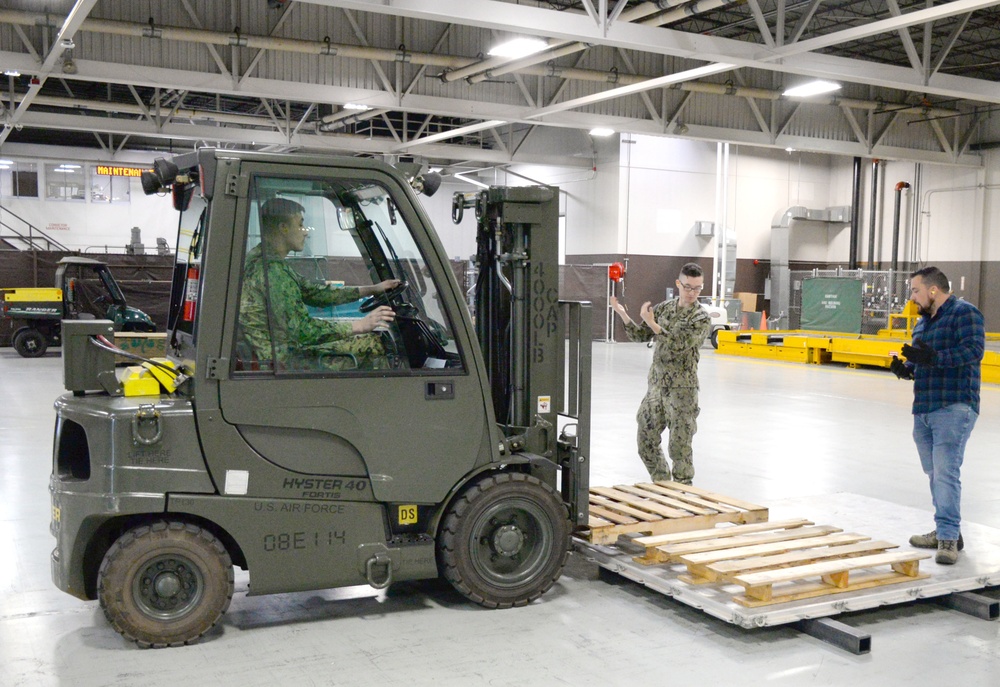This image captures a detailed scene inside a warehouse-like facility, showcasing three individuals engaged in collaborative work around a dark green forklift. The scene is set against a backdrop featuring a brown and white color-striped wall with industrial metal beams and various ducts and pipes along it. The warehouse floor is glossy and paved, and overhead, lights hang from the white industrial ceiling.

The focal point is a dark green forklift, marked with "Hyster 40 Fortis US Air Force 08E114" on the door and "4000LB CAP" on the elevator. The forklift is operated by a young man in army fatigues with short brown hair, who is maneuvering the vehicle to lift a metal platform supporting two wood pallets.

In the foreground, directing the forklift operator, is a man with short brown hair, black glasses, and combat fatigues on the left side of the frame. He holds his hands up, providing guidance. On the right side of the frame stands another man, dressed in blue jeans, brown boots, a blue flannel shirt, black gloves, and white earplugs; he has a short brown beard and short black hair. This man is also gesturing towards the forklift, aiding in the positioning of the pallets.

In the far right background, a piece of yellow machinery sits with a fenced area behind it, adorned with a green flag. This setting provides a clear picture of teamwork and precision in an industrial working environment.